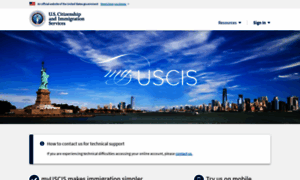The image is a slightly cut-off screenshot of a section from a website, with the lower portion missing. The text within the image is significantly blurry. At the top, there is a light gray bar spanning the width from left to right. On the left side of this bar, there is blue text accompanied by an icon of the American flag positioned to its left.

Below the gray bar, there is a white bar also stretching the full width of the image. Positioned slightly inward from the left edge of this bar is a circular logo, followed by three small lines of blue text, possibly indicating the website's address or name. On the right side of this white bar, there appear to be a login button and a resources button.

Underneath the white bar is another section featuring an image, which contains white text in the center that reads "MyUSCIS".